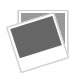The image is of a detailed war miniature, likely made of metal, depicting a German soldier from either World War I or World War II. The soldier appears in a long, heavy greatcoat, typical of those worn by Germans in Russia, and a German-style helmet. His face is indistinct, possibly melted or blurred, and he also seems to be wearing gloves. This miniature, which may resemble a sculpture or ceramic figure, shows the soldier standing on a diorama base that represents a bombed-out urban setting. The base features a sidewalk with a collapsed building, piles of bricks, and other debris scattered around. To one side of the soldier, there's a row of objects resembling upside-down skateboards or possibly rail tracks, highlighting more destruction. Below the sidewalk, there's considerable debris, suggesting a severe collapse or impact, and the entire scene might be carved from a single piece of material that’s been painted a greenish color. The figure itself seems to be a separate piece, carefully detailed to enhance the overall realism and narrative of the destruction around him.